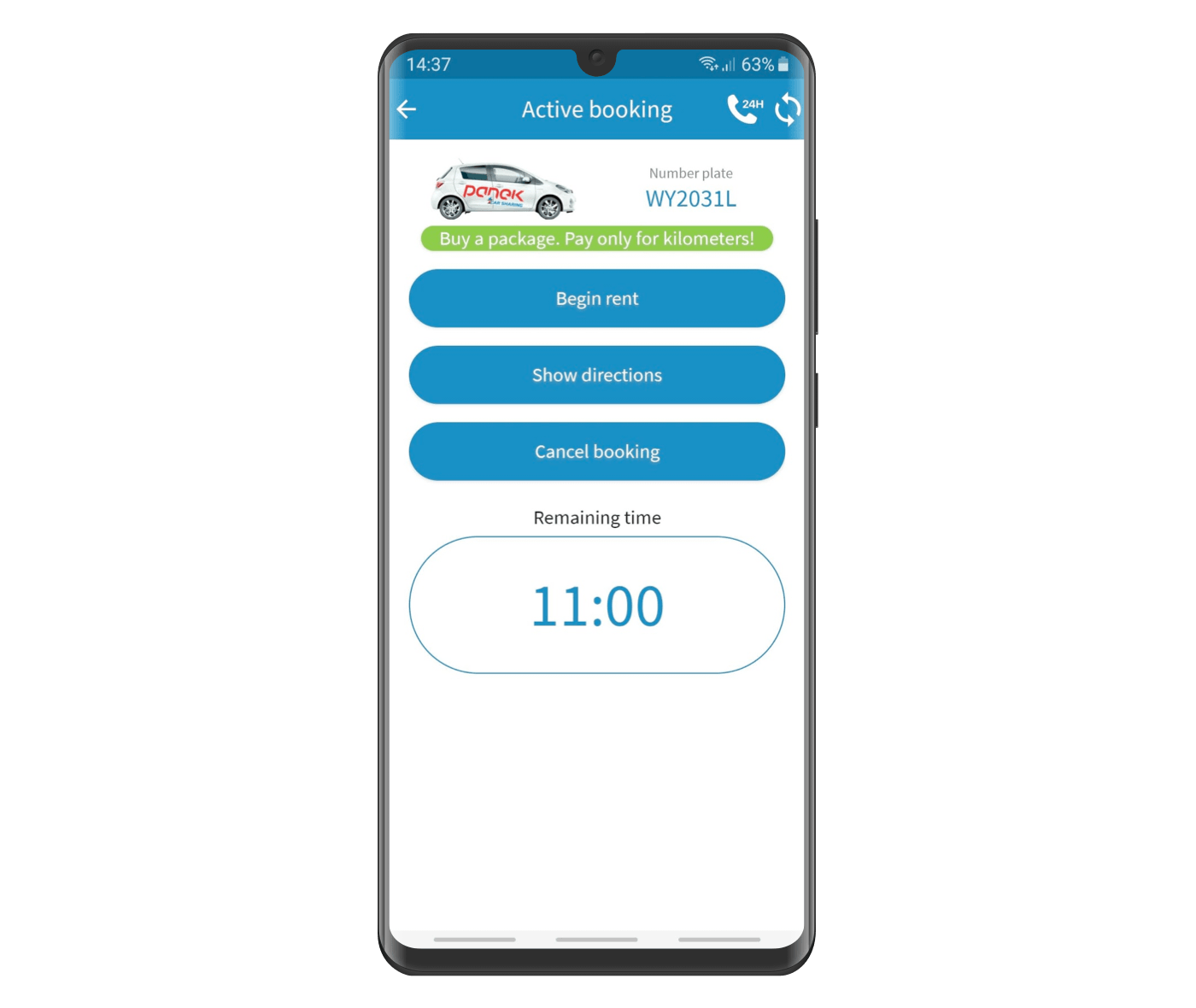The image is a screenshot of a cell phone displaying an app interface. The phone itself has a black border and physical buttons on the right-hand side: a small power button located mid-way up and a larger volume control button situated just above it.

On the phone's screen, there's a blue header at the top. In the upper left corner, the time is displayed as "14:37." The upper right corner shows Wi-Fi and data icons along with a battery life indicator at 63%.

Below the header, a white back arrow against the blue background is labeled "24-hour phone," followed by a refresh icon. The main section of the screen features an image of a vehicle with "PANEK" written in red on its side. Underneath the vehicle image, the license plate "WY2031L" is displayed. The text "Buy a package, pay only for kilometers" accompanies this information. 

Below the vehicle details are three interactive buttons labeled "Begin Rent," "Show Directions," and "Cancel Booking." At the bottom of the screen, there's a blue circle indicating the remaining rental time, currently displayed as "11:00" hours.